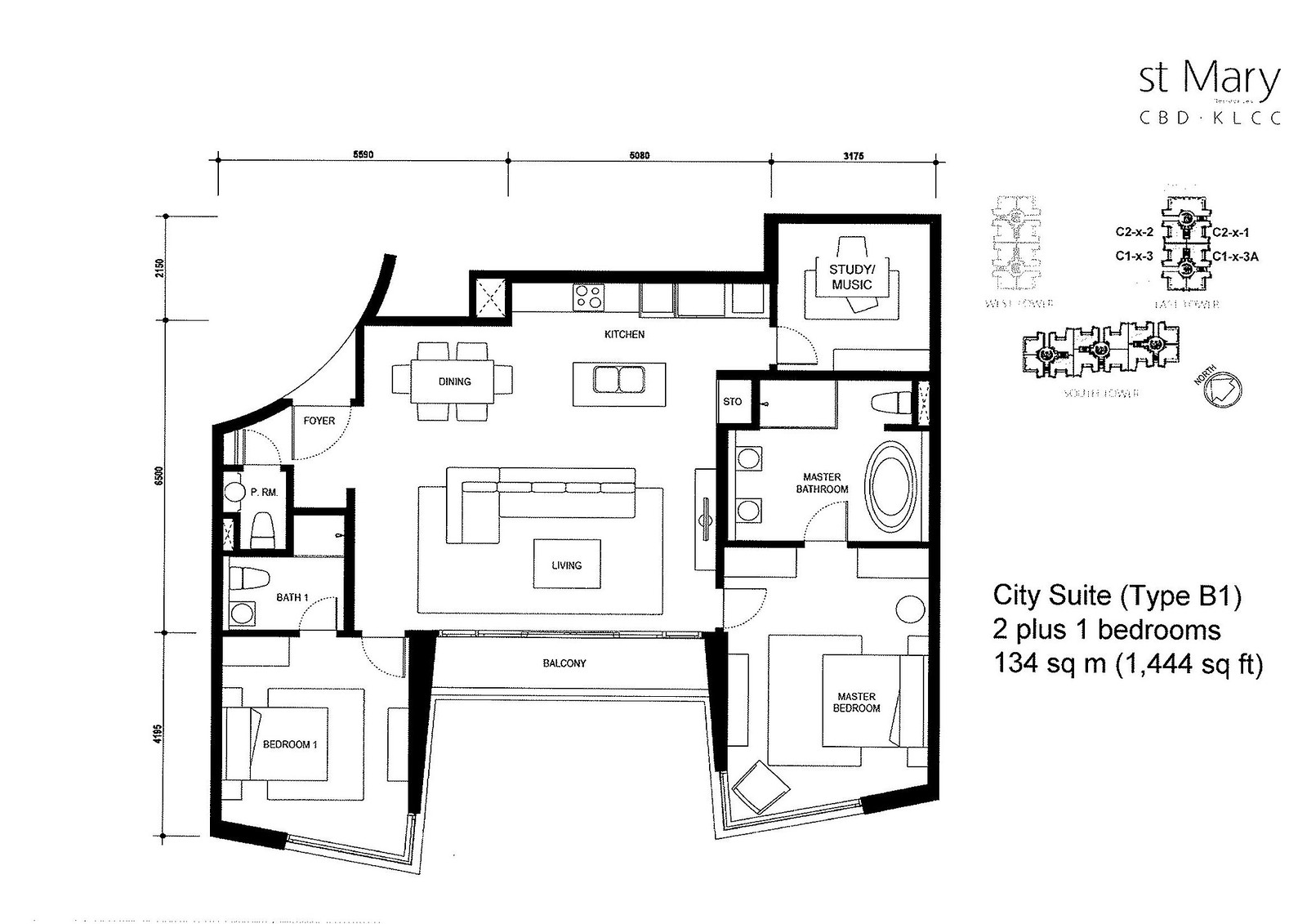In this black and white blueprint, the intricate layout of a residential property, either a home or an apartment, is meticulously detailed. Each room is precisely labeled, indicating its exact location and dimensions within the building. The blueprint is professionally drawn, using a combination of thin and bold lines to distinguish structural elements and room divisions. 

Off to the side of the blueprint, the text "St. Mary CBD KLCC" is prominently displayed, suggesting the name or location of the property. Below this, additional text indicates the specific type of unit: "City Suite (Type B1)." Details include an accommodation description of "2+1 Bedrooms," signifying two main bedrooms and an additional smaller room, potentially used as a study or guest room. The total area is noted to be 134 square meters, which is equivalently marked as 1,444 square feet.